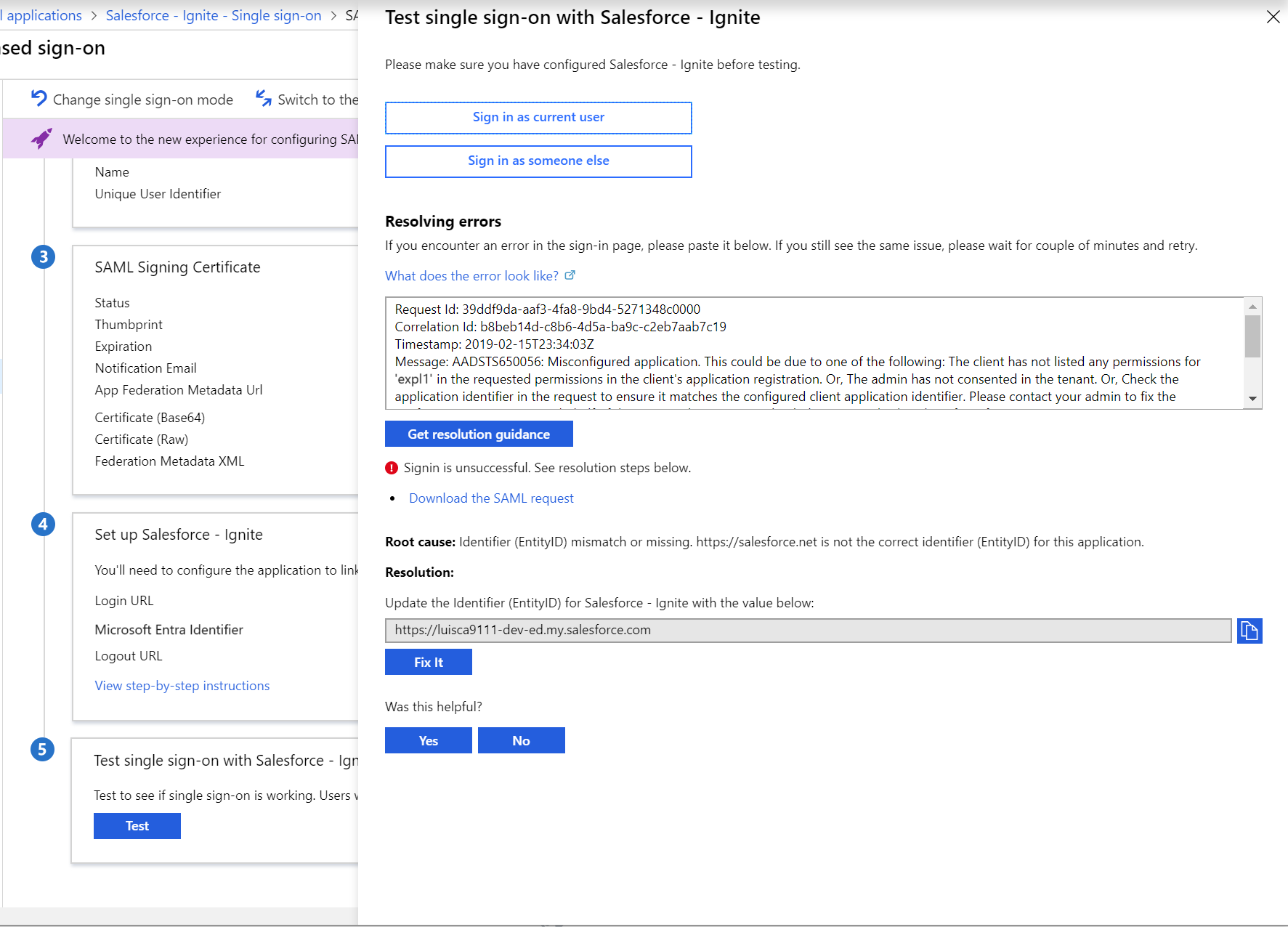Here's a cleaned-up and detailed caption for the image described:

---

The image is a screenshot of an interface from a website or application, characterized by a white background with black text and blue elements used for clickable items. At the top of the interface, there is a heading that reads "Test Single Sign-On with Salesforce-Ignite." Below the heading, a subheading advises users to "Please make sure you have configured Salesforce-Ignite before testing."

Continuing down the page, there are two prominent blue buttons with rectangular outlines. The first button is labeled "Sign in as Guest User," and the second is labeled "Sign in as Someone Else." 

Further down, the section titled "Resolving Errors" is displayed in bold text. This section provides instructions for users encountering errors on the sign-in page, advising them to paste the error message below and wait a couple of minutes before retrying. An enclosed box contains example text of what such an error message might look like.

Below the example error message, another blue button labeled "Get Resolution Guidance" is present. Beneath this button, a message explains the "Root Cause Identifier Entity ID Mismatch or Missing" and provides a website address for further information.

The next section, titled "Resolution" in bold text, instructs users to "Update the Identifier Entity ID for Salesforce-Ignite with the value below." A gray box beneath this text displays a website address. Under this box, there is a blue button labeled "Fix It."

Additionally, there are unspecified elements and information located in the left-hand column, not fully detailed in the provided description.

---

This caption thoroughly describes the visual layout and content of the screenshot, providing a clear understanding of the interface and its functionalities.